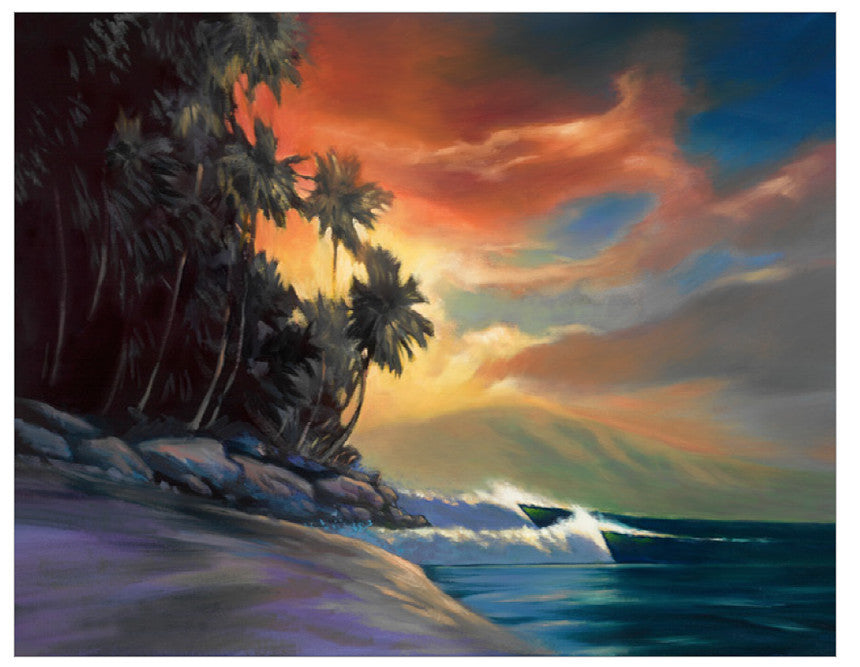This vibrant artwork depicts a serene seascape at sunset, possibly inspired by Hawaii. The left side of the painting features an array of tall palm trees of varying heights, with large rocks scattered in the foreground. The shore transitions into the beach area, washed by light blue water melding into a darker greenish-blue ocean. At the center, two white-capped waves are visibly cresting towards the shore. The right half of the image is dominated by a colorful sky, blending shades of orange, red, pale yellow, and cream, with hints of green, all centered around a setting sun peeking through streaked clouds. In the distance, a silhouette of a mountain looms against the vibrant sky. Vivid hues of blue, from dark to aquamarine, illustrate the deepening ocean waters. The painting is a harmonious blend of dark and light tones, likely achieved through acrylic or oil paints.